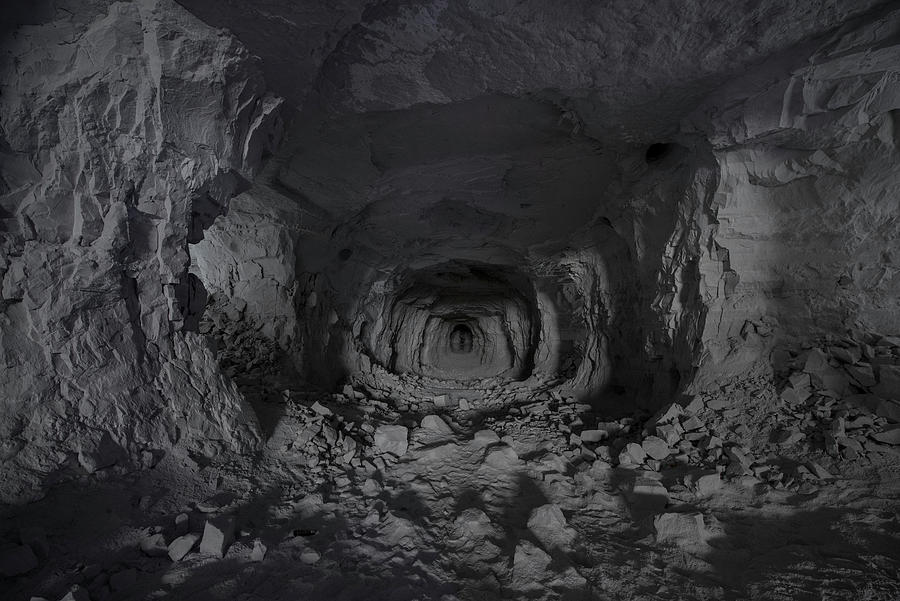The image depicts a dark, man-made tunnel that appears to be carved out of a rocky mountain, possibly for the extraction of slate or another type of stone. The tunnel extends deeply into the frame, creating a narrowing perspective much like a long hallway. This depth is accentuated by the diminishing size of the tunnel as it approaches the horizon. The scene features a clean, yet rugged environment with a variety of unique, beat-up rocks lining the ceiling and floor. The flooring is scattered with broken rocks and gravel. The overall color scheme is a blend of grayish-white tones, characteristic of a black and white photograph, but there's ambiguity whether it's actually a color photo with very low light. This tunnel, resembling a cavern or a cave with its dank and somewhat eerie atmosphere, appears both desolate and treacherous, evoking a sense of cautious exploration.